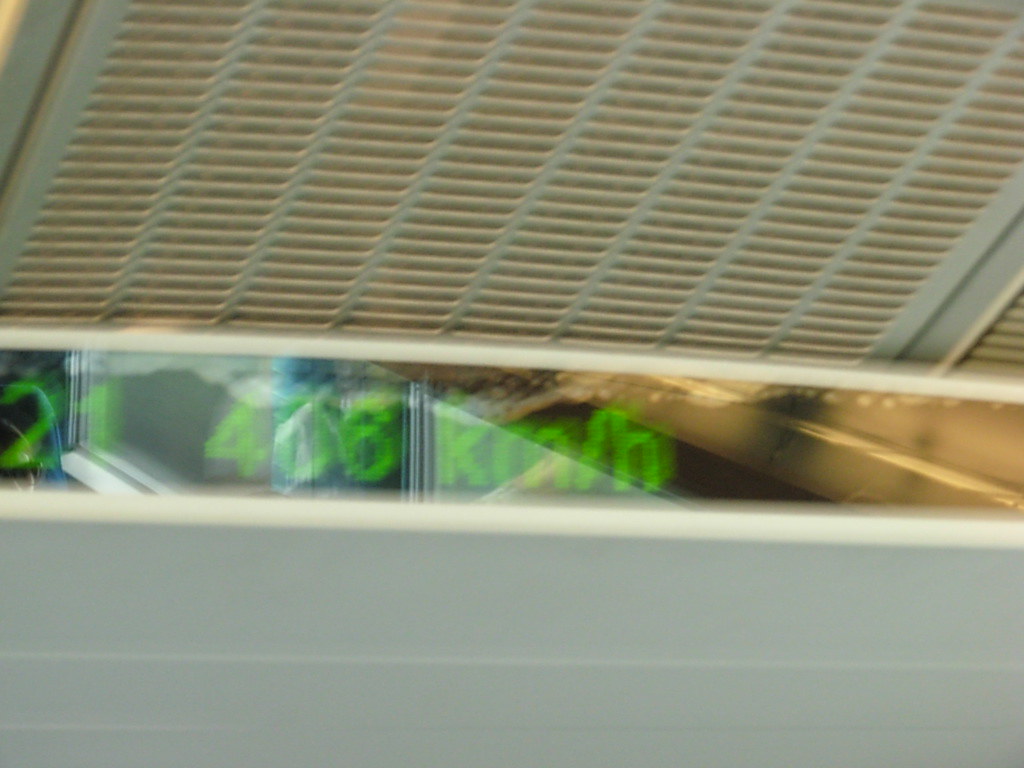The photograph is quite blurry, capturing an indistinct scene. At the base of the image, there's a gray rectangular shape. Above this, a thin off-white line can be seen, separating the gray rectangle from a black display screen positioned above. The screen exhibits a mix of green digital lettering and numbers, although the characters are partially obscured by a light glare. Above the display, there's a close-up view of a slightly off-white grate-like object, with visible graininess and blur making it challenging to discern its purpose. The image overall is marred by streaks of light, adding to the difficulty in identifying specific details.